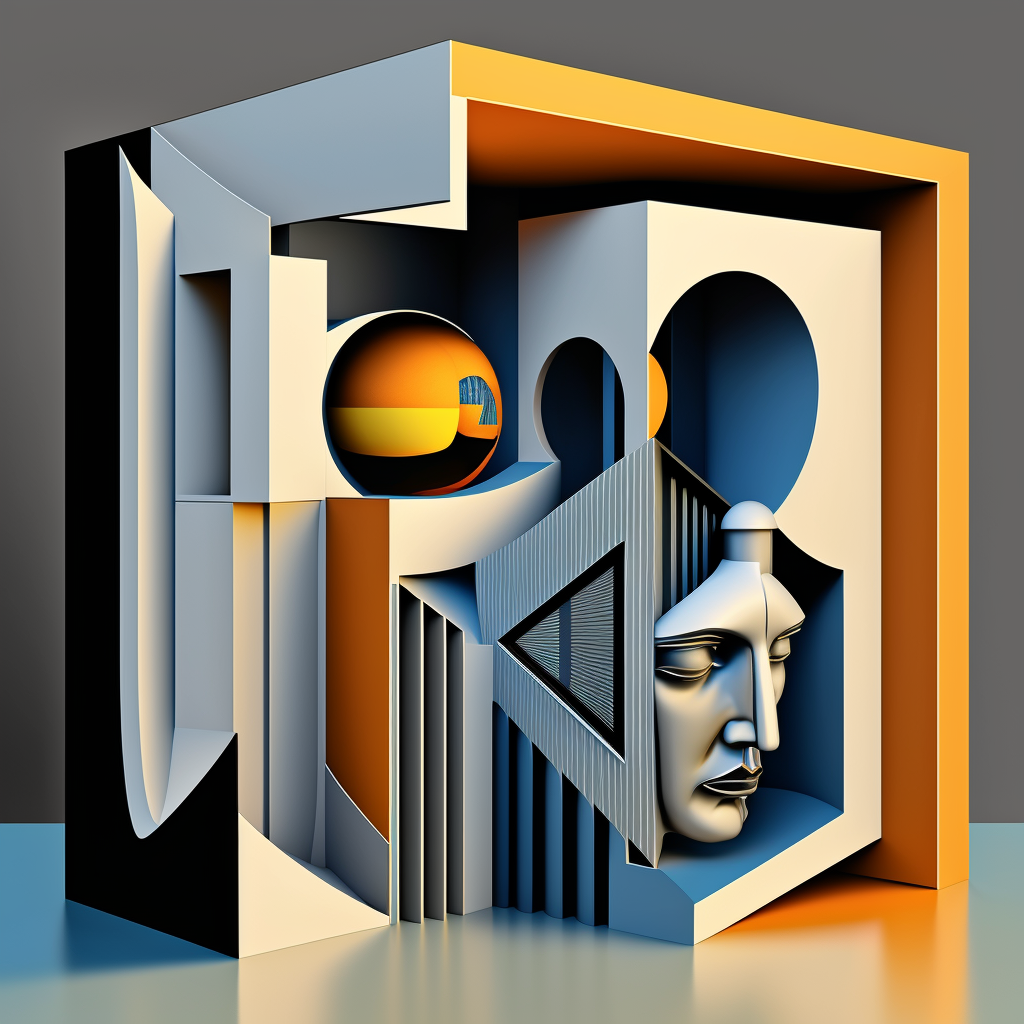This abstract art piece features a complex composition centered around an open, multi-layered cube. In the bottom right-hand corner of the inner cube, a discernible face is visible. This inner cube exhibits shades of blue and gray with additional black and white shading on the left side. The face is adorned with various geometric shapes, including a cylinder, a half-circle, and a sideways staircase. At the top of these shapes sit a yellow half-circle and a blue, yellow, and black shaded orange sphere. The outer cube, tinged in bright orange and yellow, further intensifies the intricate design with additional rectangular and circular cutouts leading from the inner to the outer sections. The entire composition is a vivid amalgamation of shapes and colors, making the face inside the cube the central, recognizable element amidst the surrounding abstract forms.